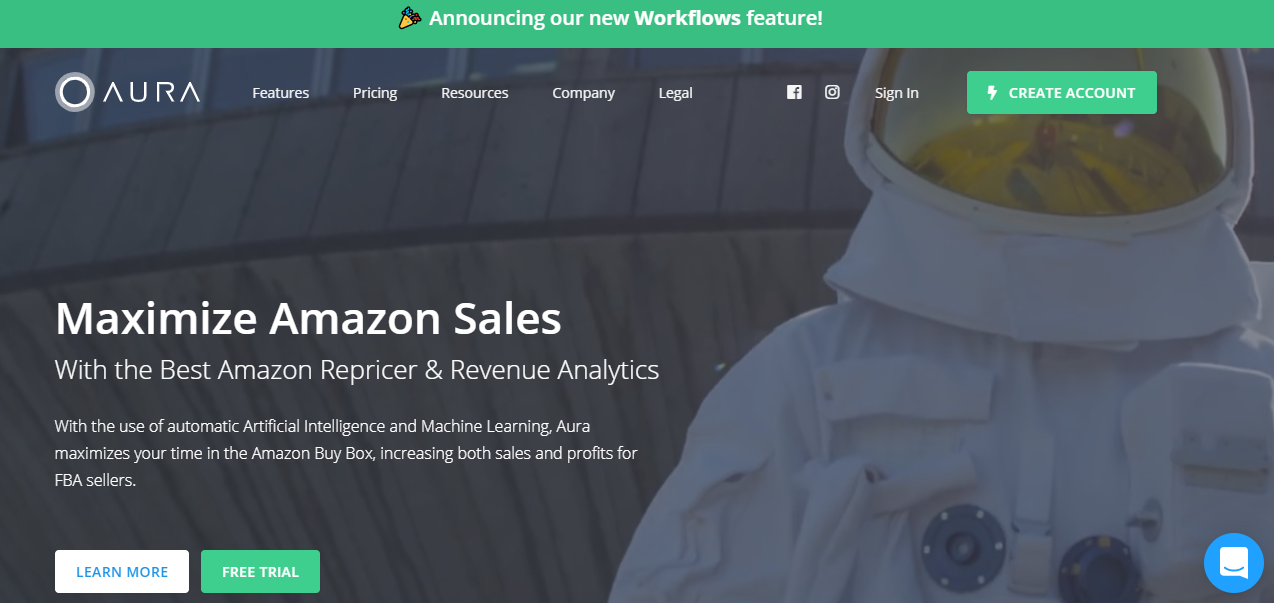On the website, the top border is green, and in the center, white text announces "Our New Workflows Feature!" Below this, a colorful cone with blue and red hues stands prominently. Further down, a white bar at the top features white columns labeled "Features," "Pricing," "Resources," "Company," and "Legal." To the right of these columns, icons for Facebook, a camera, a sign-in button, and a green "Create Account" button in white text are visible. 

The main section of the webpage has a gray background. On the right-hand side, there's an image of a white spacesuit, complete with a clear-front helmet, but no person inside. On the left-hand side, white text reads: "Maximize Amazon sales with the best Amazon repricer and revenue analytics using automatic artificial intelligence and machine learning. Aura maximizes your time in the Amazon Buy Box, increasing both sales and profits for FBA sellers." Below this, there are two call-to-action buttons: a white "Learn More" button and a green "Free Trial" button.